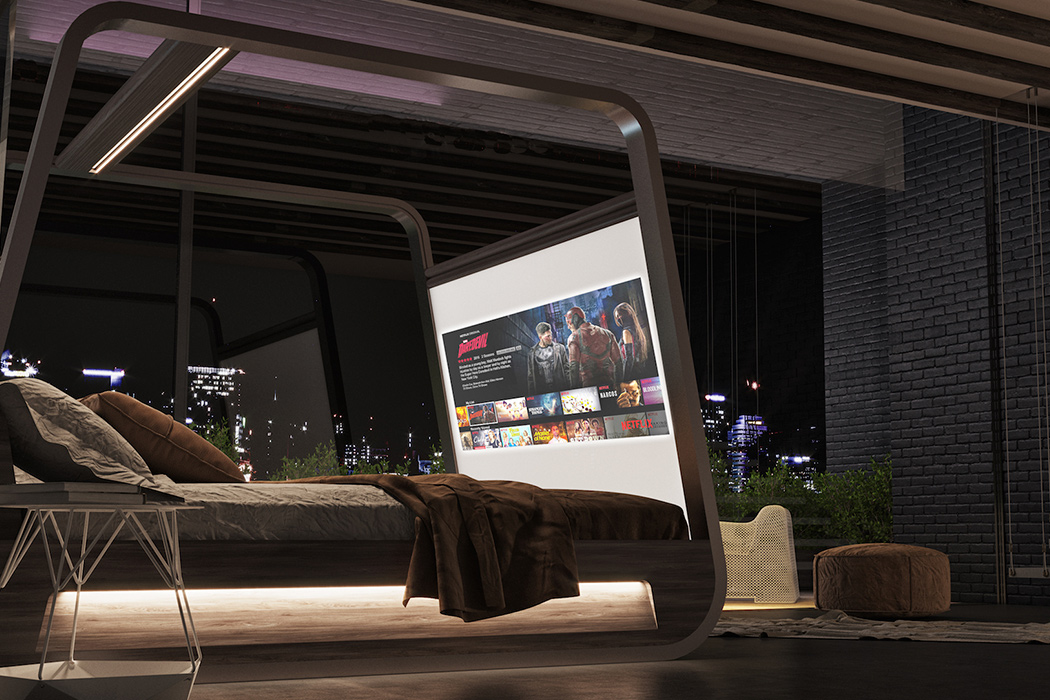This photograph showcases an ultra-modern bedroom featuring a minimalist and polygon-shaped bed frame with rounded metal edges. Built into the bed frame is a gigantic flat-screen TV displaying Netflix, currently set on Daredevil. The bed is impeccably made with brown pillows, a brown blanket, and is complemented by a light brown footstool adorned with an assortment of plants. Above the bed is a tiny, fixated light that provides a sleek overhang illumination. Through the large floor-to-ceiling glass window behind the bed, an illuminated cityscape can be seen, accentuating the room's modern, futuristic atmosphere. The room is completed with black-painted brick walls and exposed ceiling beams, creating a sophisticated and stylish master bedroom ambiance.